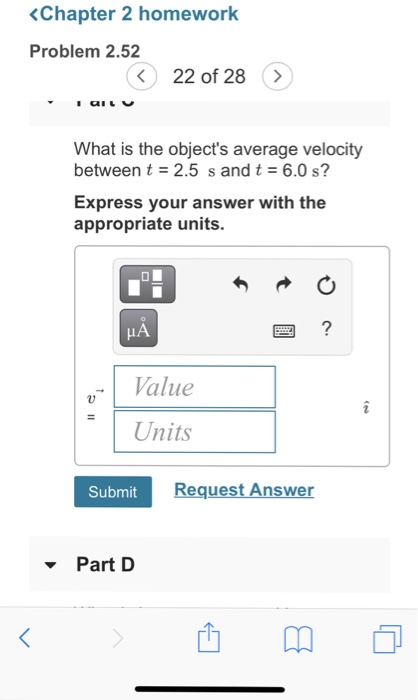The image depicts a screenshot from a white-background educational app, specifically displaying Chapter 2 homework. "Chapter 2 Homework" is written in blue at the top. Grey text below indicates "Problem 2.52," and there are navigation arrows in circular icons to the left and right, marked "22 of 28."

The problem on the screen asks: "What is the object's average velocity between t = 2.5 s and t = 6.0 s? Express your answer with the appropriate units." Below the question, there are input fields: one for "Value" and one for "Units," both highlighted in blue rectangles. Additional navigation includes a back arrow and a forward arrow.

The interface also features a virtual keyboard, a question mark icon, and buttons for "Submit" and "Request Answer." A drop-down menu labeled "Part D" is visible, along with blue icons for sharing and bookmarking the content.